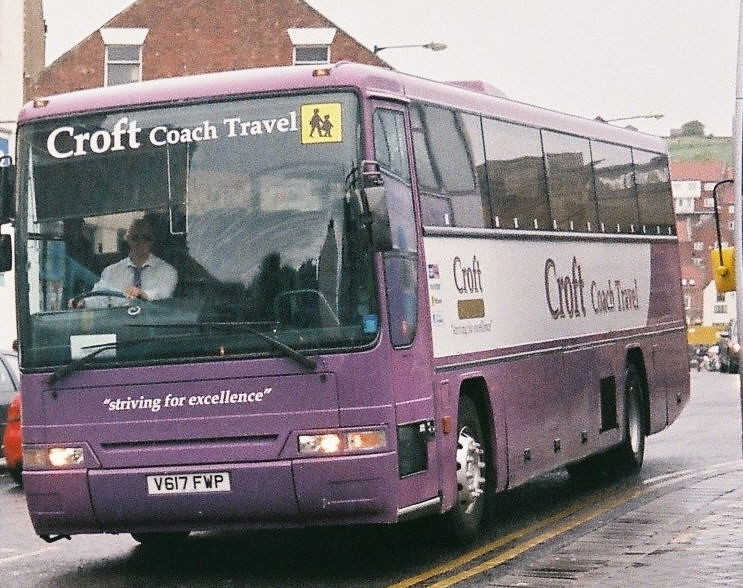The image captures a daylight, color photograph of a coach bus, primarily purple with white livery, situated in a town setting. The bus is positioned front and slightly to the sides, showcasing both its front and left side. Prominently displayed above the large front window is the text "Croft Coach Travel" in white, accompanied by a yellow square depicting two black human figures, likely an adult and a child. Below the windshield wipers, the bus features the quote "Striving for Excellence" in white text. Seated behind the steering wheel is a driver wearing dark sunglasses, a white collared shirt, and a blue tie. The license plate reads V617FWP, indicative of a European, likely UK, origin. The side of the bus features additional white and gold text stating "Croft Coach Travel," however, some smaller details are indistinguishable due to image quality. The surrounding scene includes brick buildings and a green hillside in the background, along with a sidewalk in the foreground, suggesting the bus is on a plain street within a town. The weather appears to have been wet recently, as evidenced by smears on the windshield from the wipers.